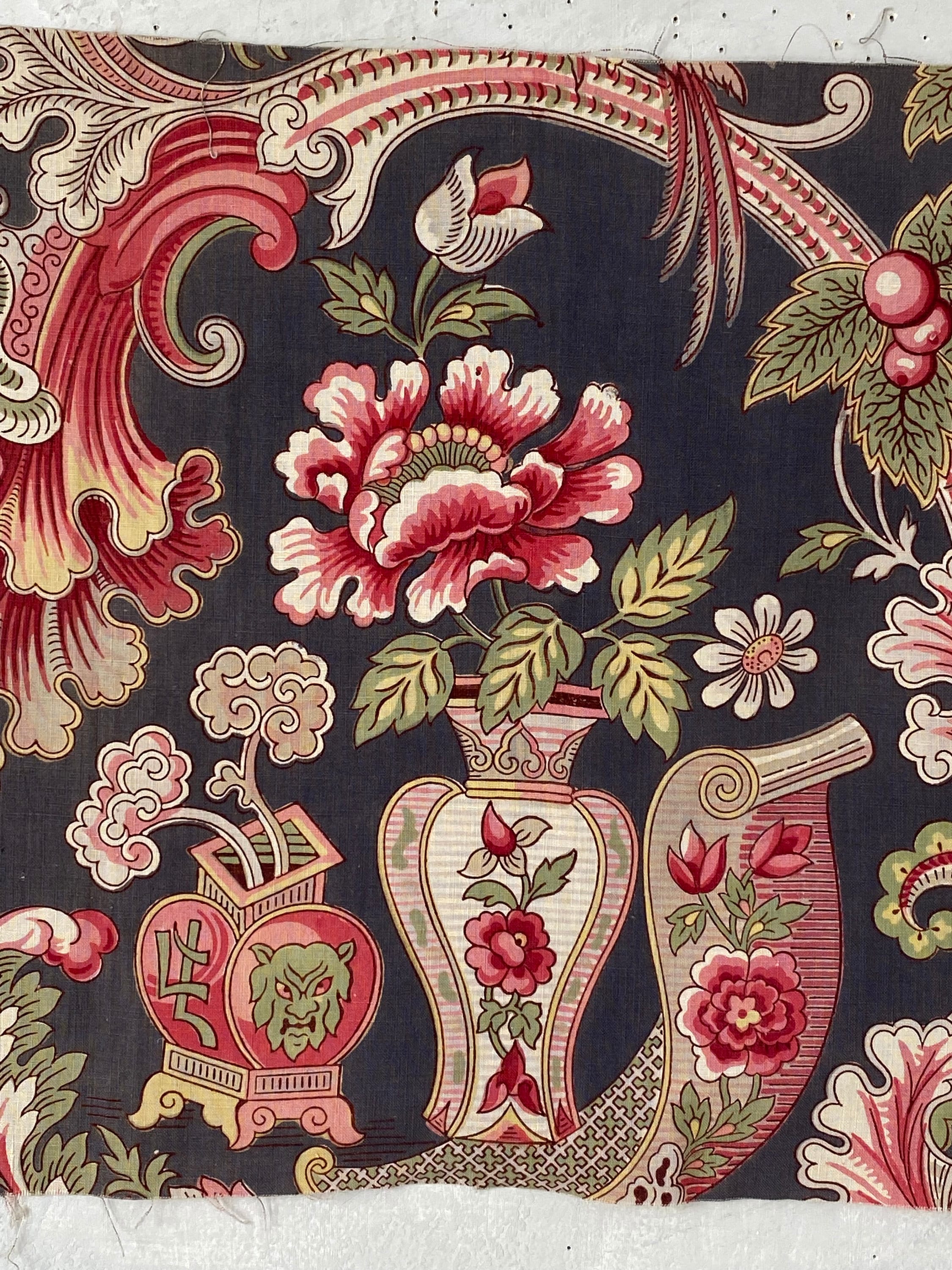This intricate image seems to be a detailed representation of a patterned fabric or wallpaper, reminiscent of designs from the 18th or 19th century, possibly akin to those by William Morris. The fabric features a striking black background adorned with vibrant colors including red, pink, white, and green. Central to the design are two vases: the first vase, white and pink, is filled with an elaborate bouquet of red, pink, and white flowers with green leaves. The second vase, intriguing in nature, showcases a green monster face along with an oriental symbol, and has light beige and pink flowers emerging from it. 

Scattered throughout the fabric are additional floral elements, including delicate designs of green leaves and red berries, likely cherries, especially noticeable in the upper right-hand corner. The entirety of the fabric is completed by ornate swirls and decorations, including fleur-de-lis patterns, enhancing its elaborate and antique look. The overall impression is bordered by a small white trim at the bottom and a grayish trim with subtle holes at the top, creating a visually appealing frame for the intricate designs within.